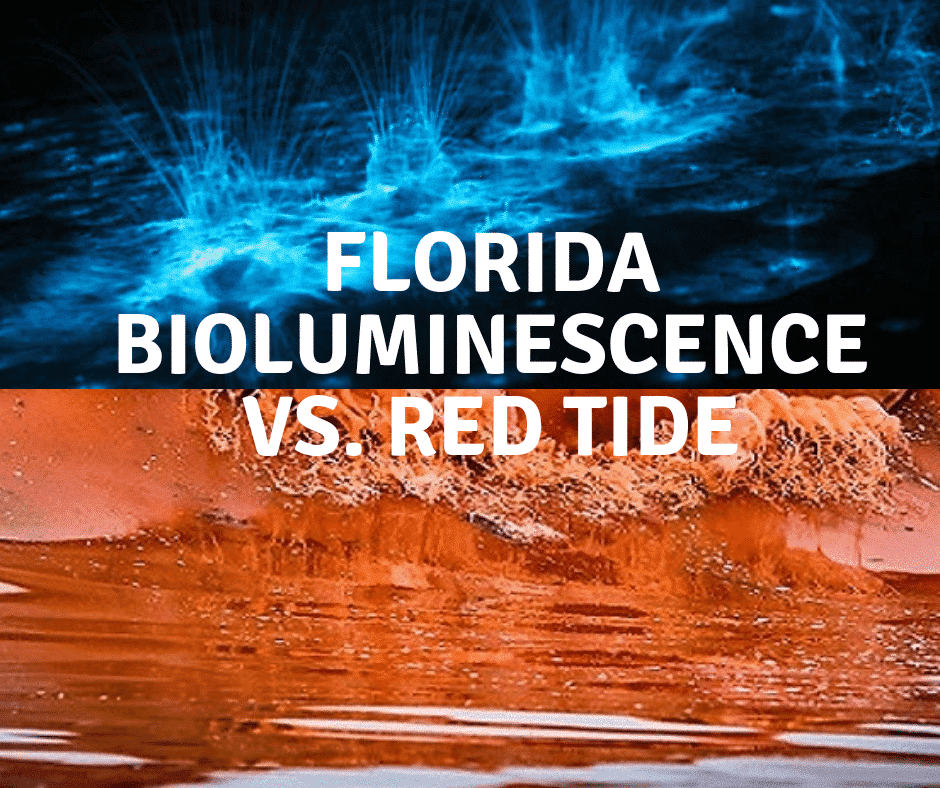The image is divided into two main sections, separated by a horizontal line, forming a square format. Both sections feature bodies of ocean water but with dramatically different colors and phenomena. The top section, which is narrow and wide, showcases a dark blue ocean labeled "FLORIDA BIOLUMINESCENCE" in bold, all-caps white sans serif font. This section is tinted a fluorescent blue and includes three areas where water splashes up, creating an eerie, bluish glow that appears almost supernatural. Below it, the bottom section is labeled "VERSUS RED TIDE" in the same bold, white sans serif font. This section displays a stark red ocean, with a central splash of water resembling red paint or foam, set against shiny red waves. Both natural phenomena are vividly captured, emphasizing the striking contrast between the mystical blue bioluminescence and the alarming red tide.